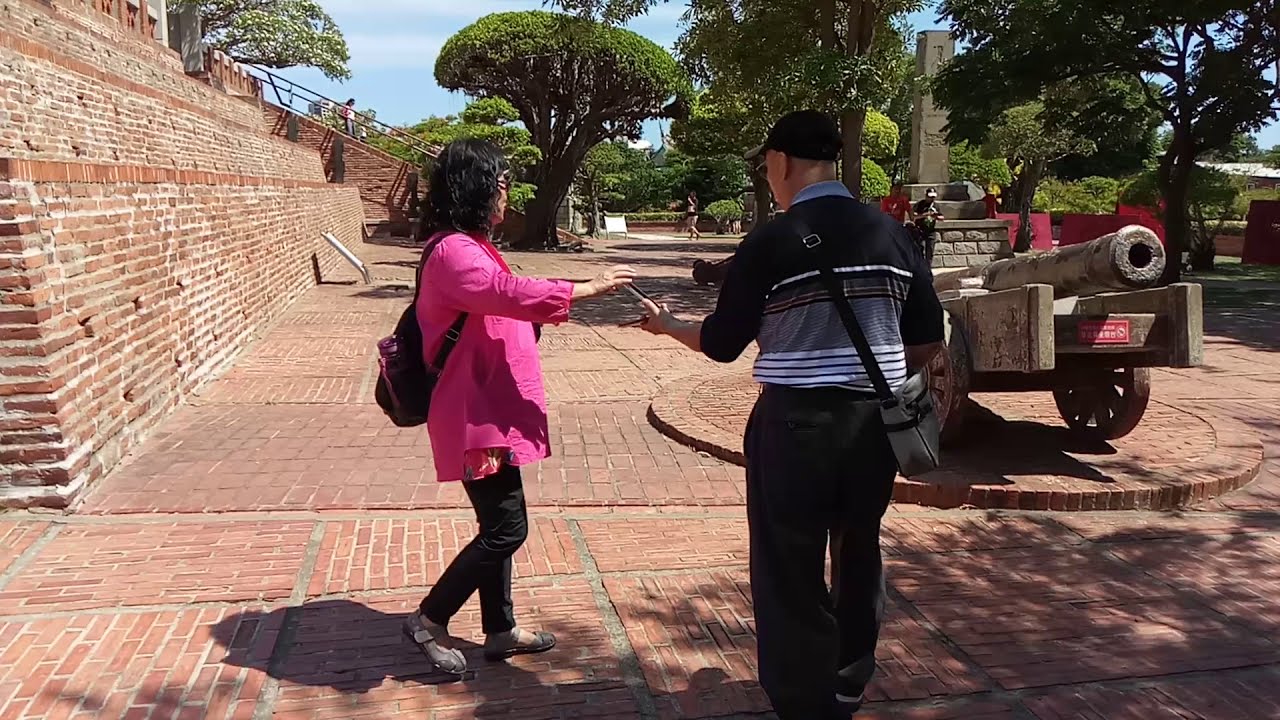The image captures a horizontally aligned, ground-level shot of a well-maintained historical site. In the foreground, a man and a woman are walking on a brick walkway, visible from behind. The man, wearing a black baseball cap, glasses, a black, white, and gray-striped long-sleeved shirt, and black pants, has a gray bag with a black strap slung over his shoulder. He appears to be handing something to the woman beside him. The woman, seen from the side, wears a long-sleeved dark pink shirt, black pants, and light brown sandals, her small black backpack hanging on her back. Both individuals are elderly. To their right, an ancient cannon, likely several hundred years old, is displayed on a wooden frame with two wheels, accompanied by an unreadable red plaque. Surrounding them is a red and brown bricked area, with a tall, aged brick wall to the left and a tiered brick system leading up to a large building partially visible in the distance. Manicured trees are scattered throughout the background, along with a brick staircase. The sky above is mostly blue with a few white clouds. The overall scene suggests a peaceful visit to a historical landmark, with the cannon adding a focal point of historical significance.